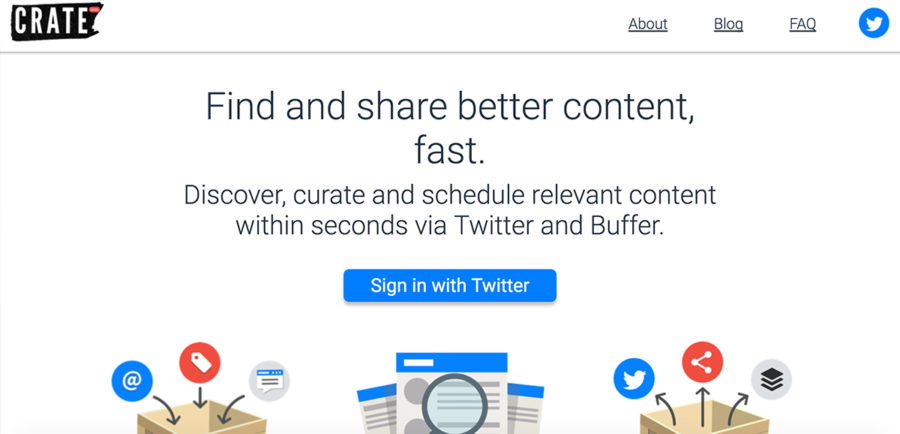This is a detailed screenshot from a website with the top banner displaying "CRATE" in all capital white letters inside a black shape. To the right, navigation links labeled "ABOUT," "BLOG," and "F-A-Q" are visible. A blue circle featuring a white bird flying to the right, symbolizing Twitter, is also present. 

Below the banner is a thin gray horizontal line separating the top section from the main content. The prominent headline reads: "FIND AND SHARE BETTER CONTENT FAST." Beneath it, a subheading says: "DISCOVER, CURATE, AND SCHEDULE RELEVANT CONTENT WITHIN SECONDS VIA TWITTER AND BUFFER." Following this is a blue rectangle with white lettering that invites users to "SIGN IN WITH TWITTER."

The bottom section of the image contains partially visible illustrations. The first illustration depicts a box receiving inputs from three symbols: an at-sign (@), a price tag, and a text bubble. The second illustration shows three pieces of paper, likely representing curated content. The final illustration features a box with arrows emerging from it, directing towards three symbols: the Twitter bird, a share symbol, and an icon resembling three stacked squares, suggesting content distribution and management.

The entire image is devoid of photographic elements and human figures, focusing solely on graphical and textual information. It is wider than it is tall, contributing to a broad layout design.